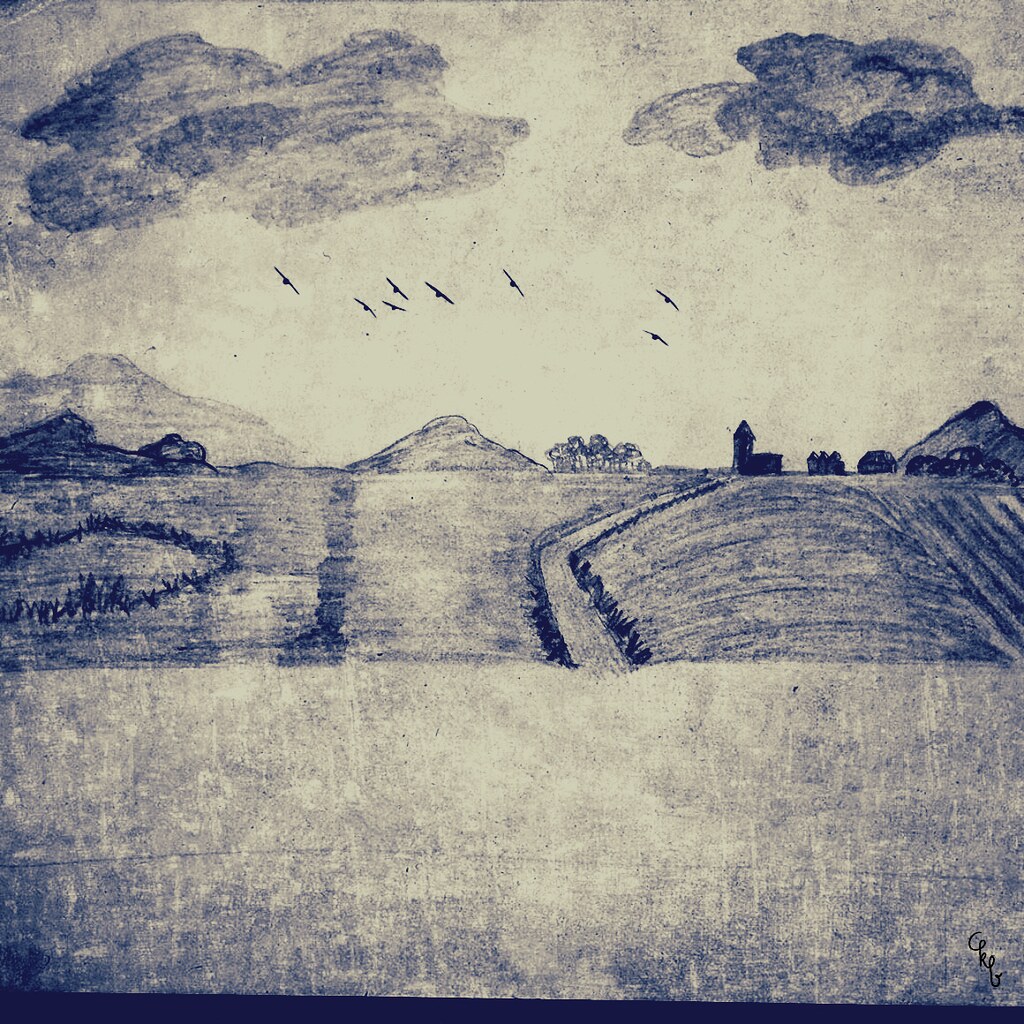This intricately detailed landscape drawing, created in varying shades of gray and black, is set against an off-white, ecru background, likely achieved using charcoal or pencil. The scene captures a serene and expansive view, characterized by a balanced composition and fine attention to detail. 

In the top portion of the frame, two clouds float gracefully; the one on the left dominates in size, while the smaller cloud on the right complements it. Below these clouds, a formation of birds soars towards the right, adding a sense of motion to the tranquil scene. 

To the left, the rugged end of a sprawling mountain range starts the visual journey. Moving towards the center, a smaller, more isolated mountain rises subtly. This middle ground leads the eye to the right, where a cluster of animals can be seen resting on a mountain slope, evoking a pastoral stillness.

Further to the right, a picturesque church with a tall, elegant steeple stands prominently, suggesting a point of community or refuge. Surrounding the church, smaller homes nestle closely, forming a quaint village scene.

Descending from this village, the land slopes gently into an open, grassy area, completing the serene and idyllic landscape with a touch of rustic charm.